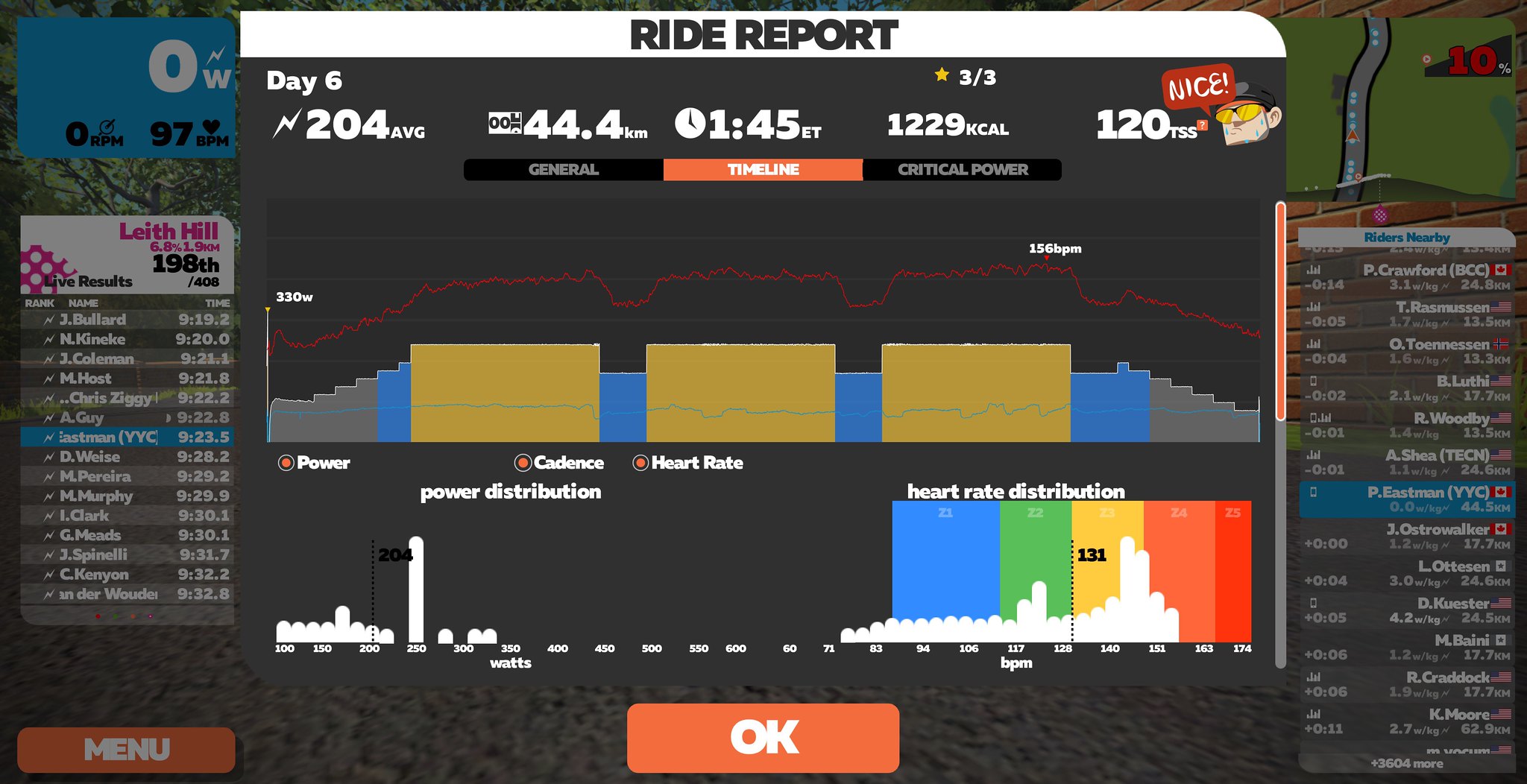The image is a screenshot from the computer game Zwift, designed for virtual cycling workouts. The interface features a charcoal gray background with primarily white text, punctuated with colorful graphical elements.

At the very top, there is a white banner with the black text "Ride Report." Directly below, it details the session specifics: "Day 6," "204 Average Watts," "44.4 Kilometers," "1:45 ET," "1,229 Kcal," and "120 TSS." Additionally, there's a fun touch with a small squirrel-shaped icon exclaiming "Nice!"

The core of the display is dominated by a combination bar chart and line chart, marked with the labels "Power," "Cadence," and "Heart Rate." These charts show various metrics, including a maximum wattage of 350, with corresponding color blocks in blue, green, yellow, orange, and deep orange indicating different ranges. Below these, the "Heart Rate Distribution" is depicted with a color bar. 

Flanking the main graph, there are lists labeled "Leith Hill" and "Riders Nearby," which include various names and numbers of other cyclists in the session. At the very bottom, menu options are available with "Menu" and "OK" buttons for navigation.